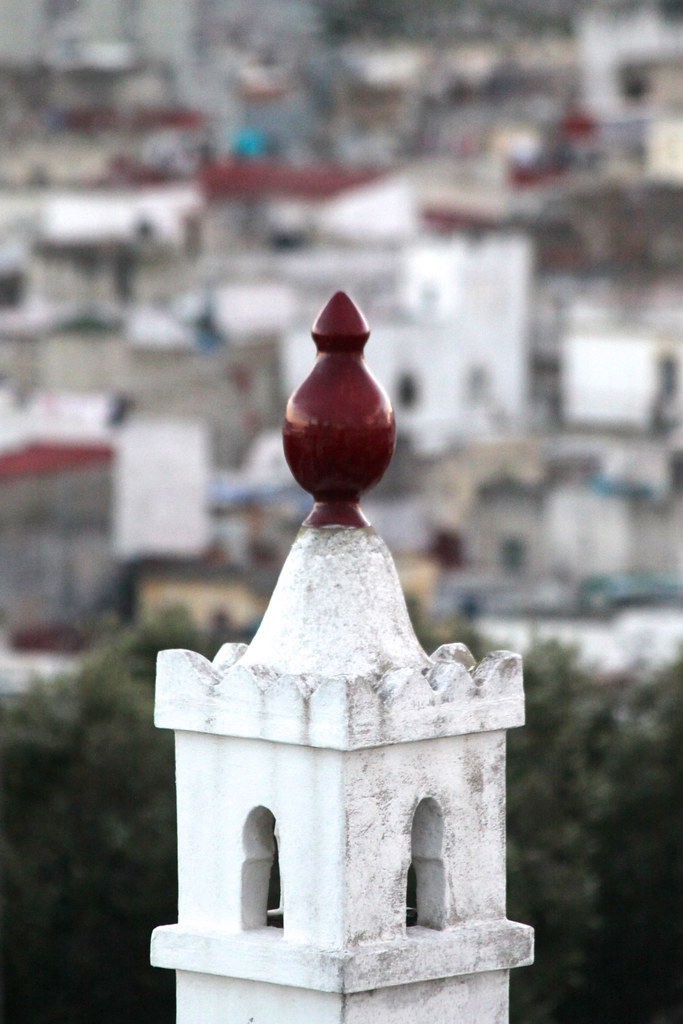This close-up photograph captures the intricate details of the top of a building, which appears to resemble a steeple or possibly the top of a rail. The structure is characterized by a square, white stone base with arched openings on at least two visible sides, and it is likely these arches are present on all four sides. Rising from the arched base is a beautifully crafted red or maroon-colored, bulbous peak that comes to a pointed conclusion. The peak's shade hints at a blend between brownish and reddish hues. The backdrop of this daytime scene is softly blurred yet reveals glimpses of a hillside dotted with more white structures that have red roofs, and small hints of black dinginess. The lower part of the image includes some greenery, likely bushes or trees. The brightness of the photograph enhances the visibility of the whites, blues, reds, greens, gray, and a touch of tan, contributing to the vibrant yet serene composition.